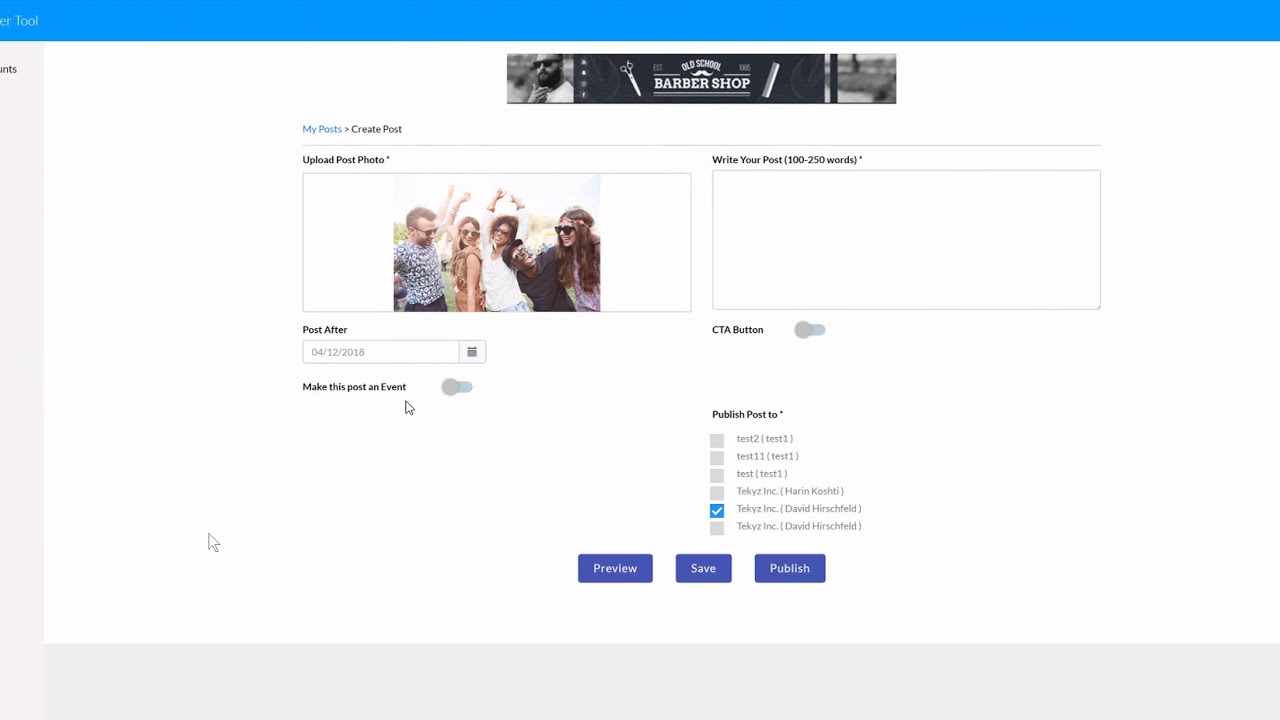This image depicts a computer screen with a user interface. At the very top of the screen, a horizontal blue banner spans the width of the page, featuring the word "TOOL" in fine white lettering positioned in the far left corner. 

Directly beneath this blue banner is another prominent banner with the title "Old School Barbershop." This banner includes a photograph on the left side of a man wearing black sunglasses and sporting a dark beard. His right hand is raised towards his chin, and he is clad in a white t-shirt, facing slightly to the front left. Within the "Old School Barbershop" banner, images of a small pair of scissors and a comb are incorporated into the logo, positioned around the text.

Below this, there is a section labeled for uploading photos, featuring an image of five people laughing and dancing, with their arms raised in the air. To the right of this image is a blank rectangle outlined in gray, possibly a placeholder for additional content.

At the bottom of the screen, there are three blue rectangular buttons with white text, labeled "Preview," "Save," and "Publish," offering options for the user to interact with or finalize their content.